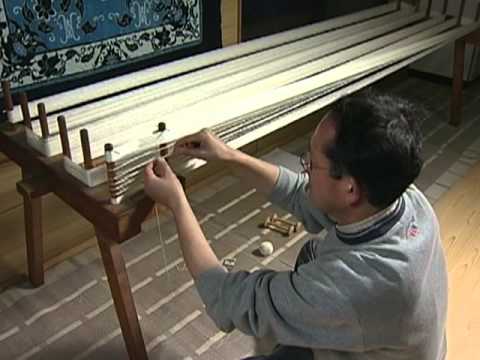In this detailed photograph, a Eurasian man is meticulously preparing a low, flat-table loom for weaving. He is crouched on the floor, focusing intently on wrapping the warp threads along the length of the wooden structure. The craftsman wears glasses and a gray sweatshirt with the sleeves pushed up to his elbows, revealing his forearms as he works. The room's floor features light brown tiles beneath a runner rug where bobbins are scattered around him. Above the loom, an elegant oriental rug hangs vertically on a tan wall, adorned with an intricate leaf motif in hues of blue, cream, and green, adding a rich backdrop to the scene. The weaver's concentrated efforts, combined with the surrounding detailed elements, highlight the dedication and artistry involved in his craft.